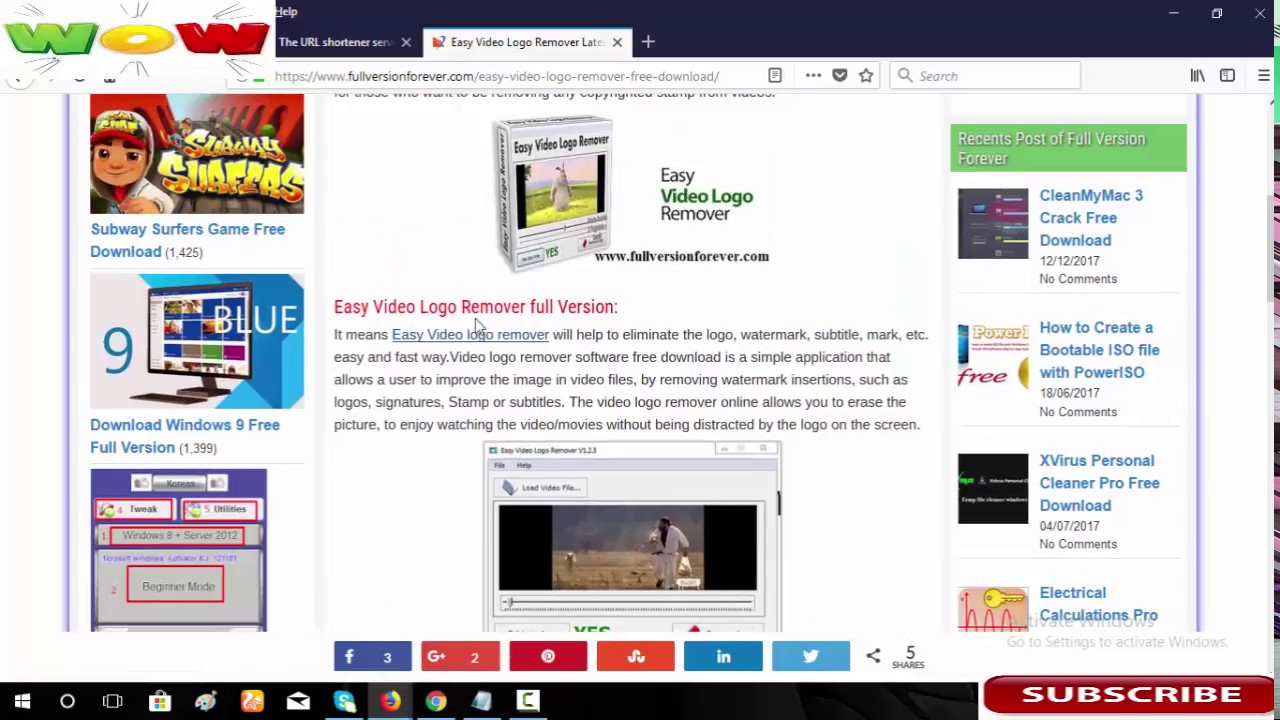This image captures a webpage from the 90s-style website fullversionforever.com, showcasing an advertisement for the software "Easy Video Logo Remover." The ad promotes the full version of Easy Video Logo Remover, emphasizing its ability to swiftly and effortlessly eliminate logos, watermarks, subtitles, and various other marks from video files. The software is accessible for free download and is designed to enhance the viewing experience by removing intrusive elements like logos, signatures, stamps, or subtitles from videos. The website itself appears to be a haven for pirated software, as indicated by a right-hand scrolling column labeled "Recent Posts of Full Version Forever," listing several software packages available for piracy, including "CleanMyMac 3, crack free download," "How to Create a Bootable ISO File with PowerISO," "X-Virus Personal Cleaner Pro free download," and "Electrical Calculations Pro."

The website layout features a left-hand column presumably offering additional software downloads, with visible items such as the "Subway Surfers game free download" and a poorly rendered image of a monitor promoting a "Download Windows 9 free full version" link. Further down, there's an indistinct image of another software product, too small to discern. The user interface suggests the individual viewing the page is operating on a pre-Windows 11 version of Windows, evidenced by the taskbar design visible at the bottom of the screen. Moreover, a distinctive overlay in the upper-left corner of the screenshot displays the word "WOW" in all caps, with a green 'W', yellow 'O', and red 'W', signifying possibly an outdated media player or graphic overlay.